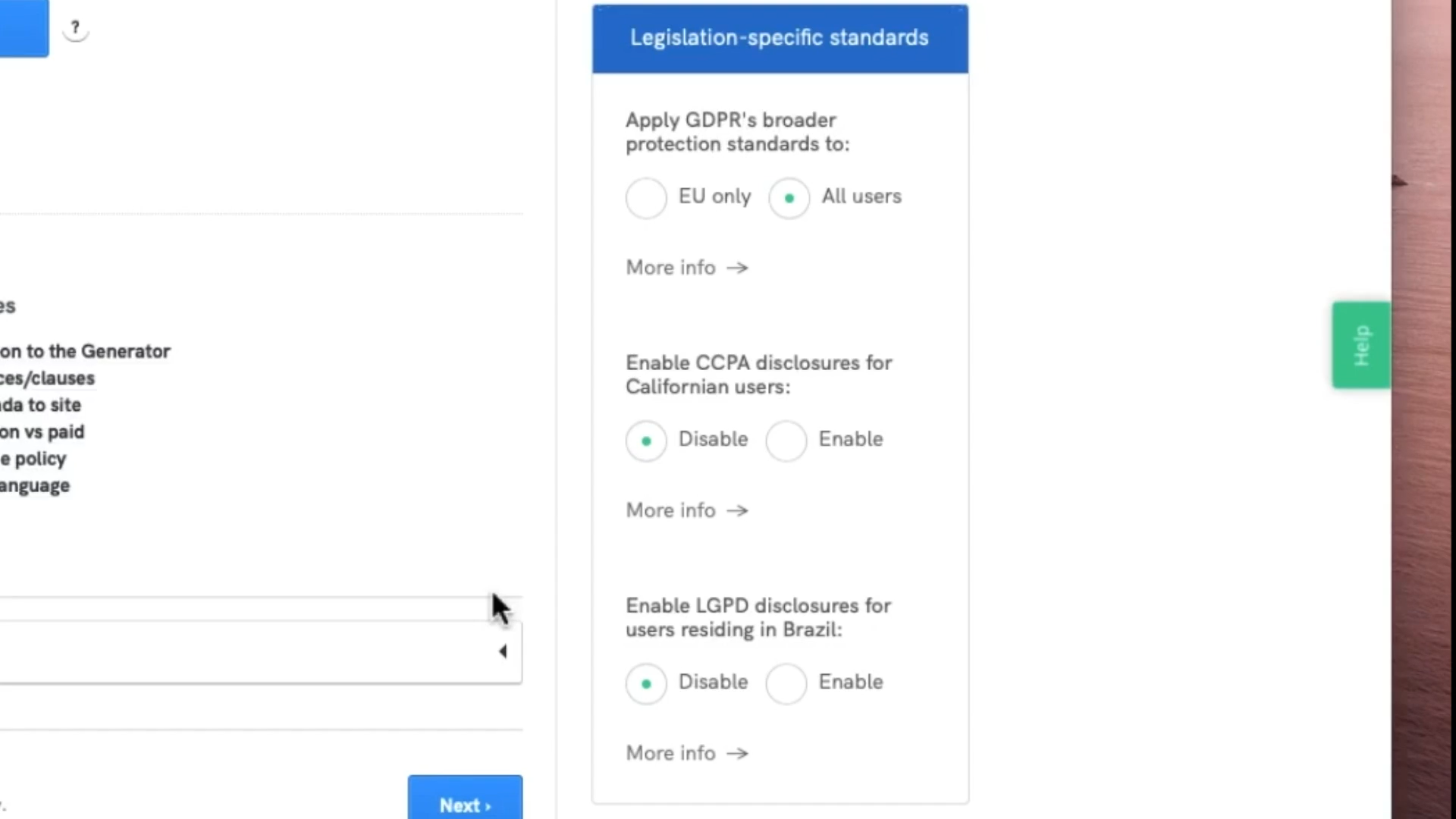Detailed Caption: 

This image depicts a help page with a primarily white background, black text, and some blue highlights. On the left-hand side, there is a vertical navigation menu. However, the text for the navigation links is cut off on the left, partially hiding their content. The visible parts of the links read: "enerator," "lauses," "ite," "aid," "olicy," and "anguage." Below these truncated links is a dropdown menu box, followed by a blue "Next" button. 

On the right-hand half of the page, there is a section headed "Legislation Specific Standards" highlighted in blue. Under this header are multiple selectable options that include "Applying GDPR's Protection Standards," "CCPA Disclosures," and "LGPD Disclosures." Additionally, at the bottom of this section, there is an arrow indicating more information is available. The company to which this help page belongs is not identified in the image.